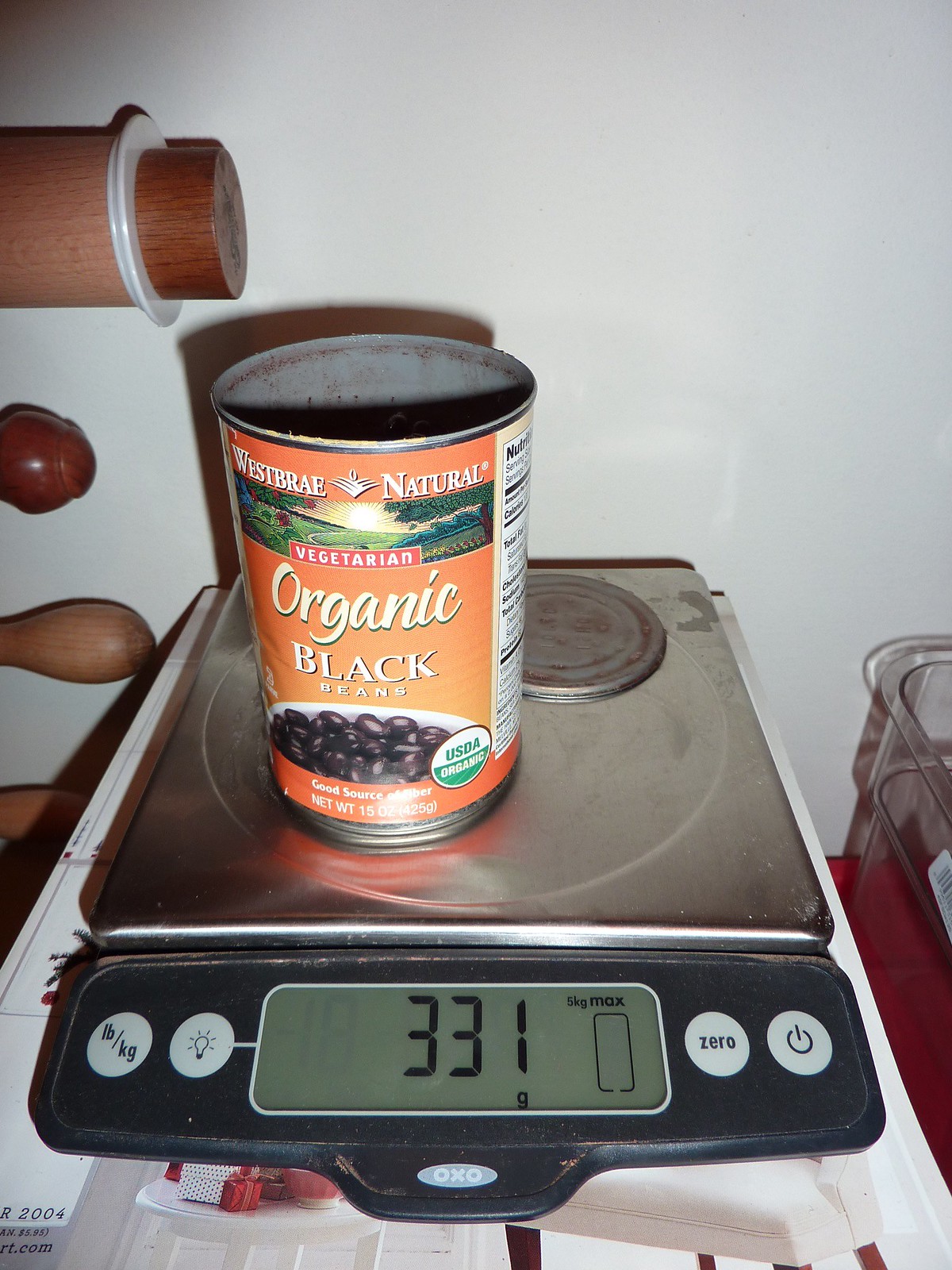This image captures a detailed scene in a kitchen setting with a digital scale prominently featured in the center. The scale, primarily white with a black interface, displays the weight "331g" on a small, slightly green digital screen. The scale includes various white buttons with black text or symbols, including a "light bulb" button, an "LB/KG" button, a "zero" button, and a power button.

Sitting atop the stainless steel platform of the scale is an open can of "West Bray Natural" brand organic black beans. The can is predominantly orange with white text and graphics, including a small white bowl filled with black beans and a barely visible nutrition label. Additional text indicates the product is vegetarian, highlighting a small farm image within a red-bordered banner.

The can's lid, also silver, is detached and placed upside down beside the can. Visible on the can's interior are dark silver surfaces with some bean residue. The background wall is pure white, with the upper right corner showing partial views of a large wooden rolling pin and other light brown wooden objects. To the right of the scale's base, there's a glimpse of a plastic container.